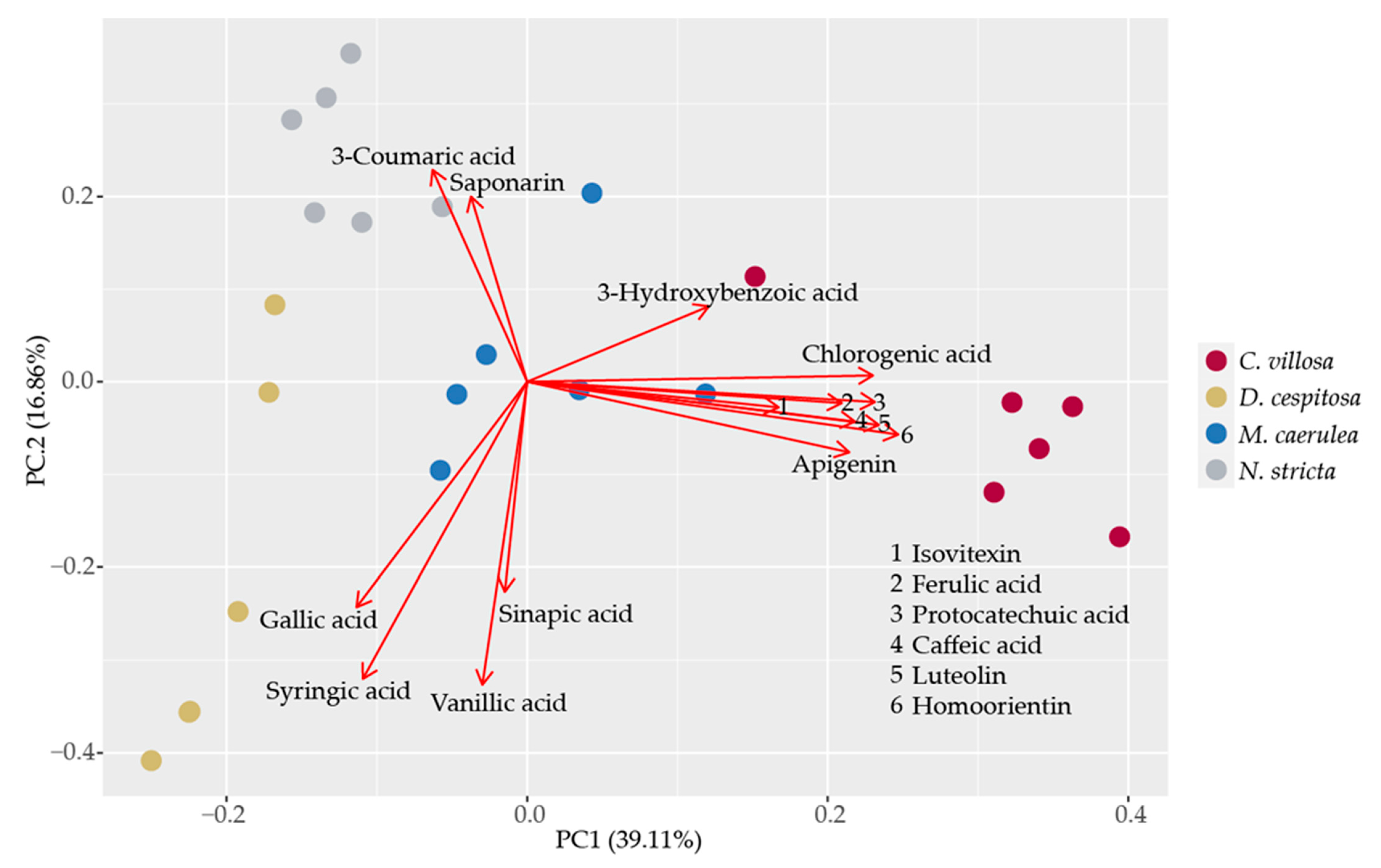This detailed caption combines the repeated and significant elements described by the different perspectives:

The image depicts a detailed scatter plot graph, likely from a scientific study in biochemistry or molecular biology. Spanning a grey grid with white lines, the graph has an X-axis labeled "PC1 (39.11%)" and a Y-axis labeled "PC2 (16.89%)". Dots in four distinct colors—red, yellow, blue, and gray—are scattered across the graph. These colors represent different groups: red for C. villosa, yellow for D. capritosa, blue for M. serousula, and gray for N. strickla, as indicated by the legend located on the right side of the image.

The graph features a series of colored dots and labels with numerous scientific terms such as 3-chlorogenic acid, siponarin, 3-hydroxybenzoic acid, chlorogenic acid, apigenin, gallic acid, syringic acid, vanillic acid, synaptic acid, isobitexin, ferulic acid, protocatechuic acid, caffeic acid, luteolin, and homoeriodictyol. Red arrows point from certain clusters of dots to these chemical names, possibly indicating significant associations or findings.

The overall design follows a coordinate system starting at (0,0) in the middle, with dots expanding outwards in an organic pattern rather than straight lines. The background is simple and grey, providing a clear contrast to the variously colored dots and helping to distinguish the different chemicals and groupings represented on the graph.